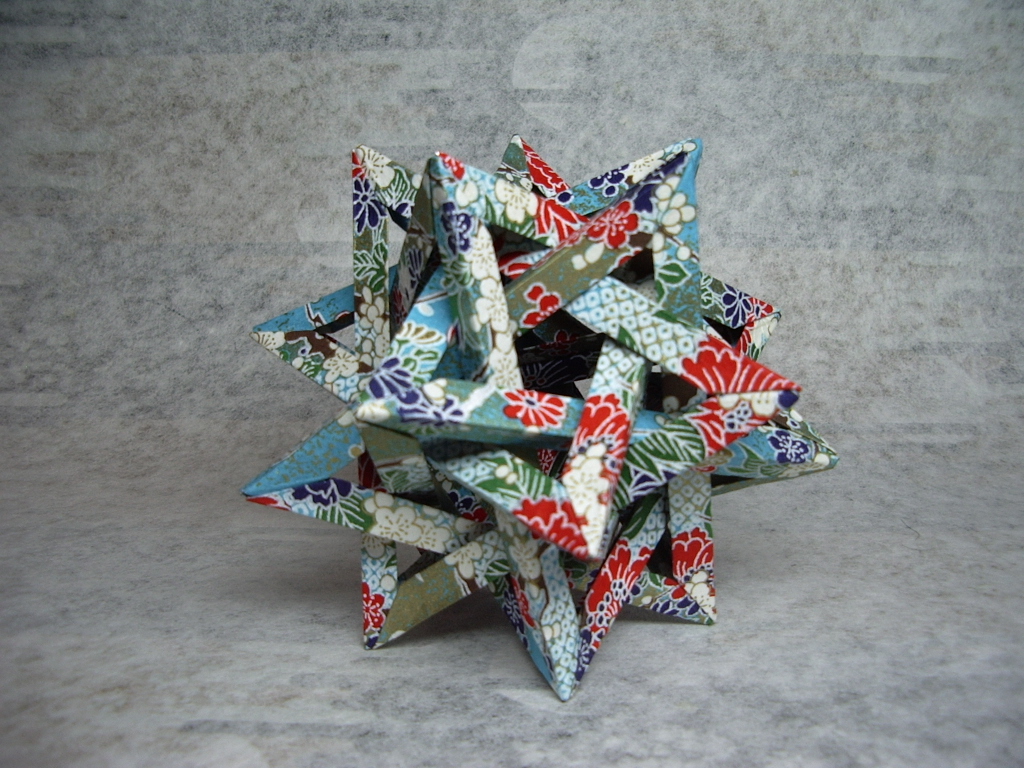This professional photograph showcases an intricate piece of origami placed against a continuous marbled gray backdrop. The origami features numerous interlocking triangular pyramids, forming a complex, multi-dimensional star-like structure. Crafted from origami paper, the piece boasts a sage green and sky blue background adorned with a vibrant pattern of white, purple, and red flowers, accentuated with darker green leaves. The paper creates an almost metallic appearance under the lighting. The origami's hollow centers allow glimpses through the intricate network of points, with thirteen visible projections adding to its elaborate three-dimensionality. The combination of the flower patterns and interwoven pyramids presents a striking and detailed visual.